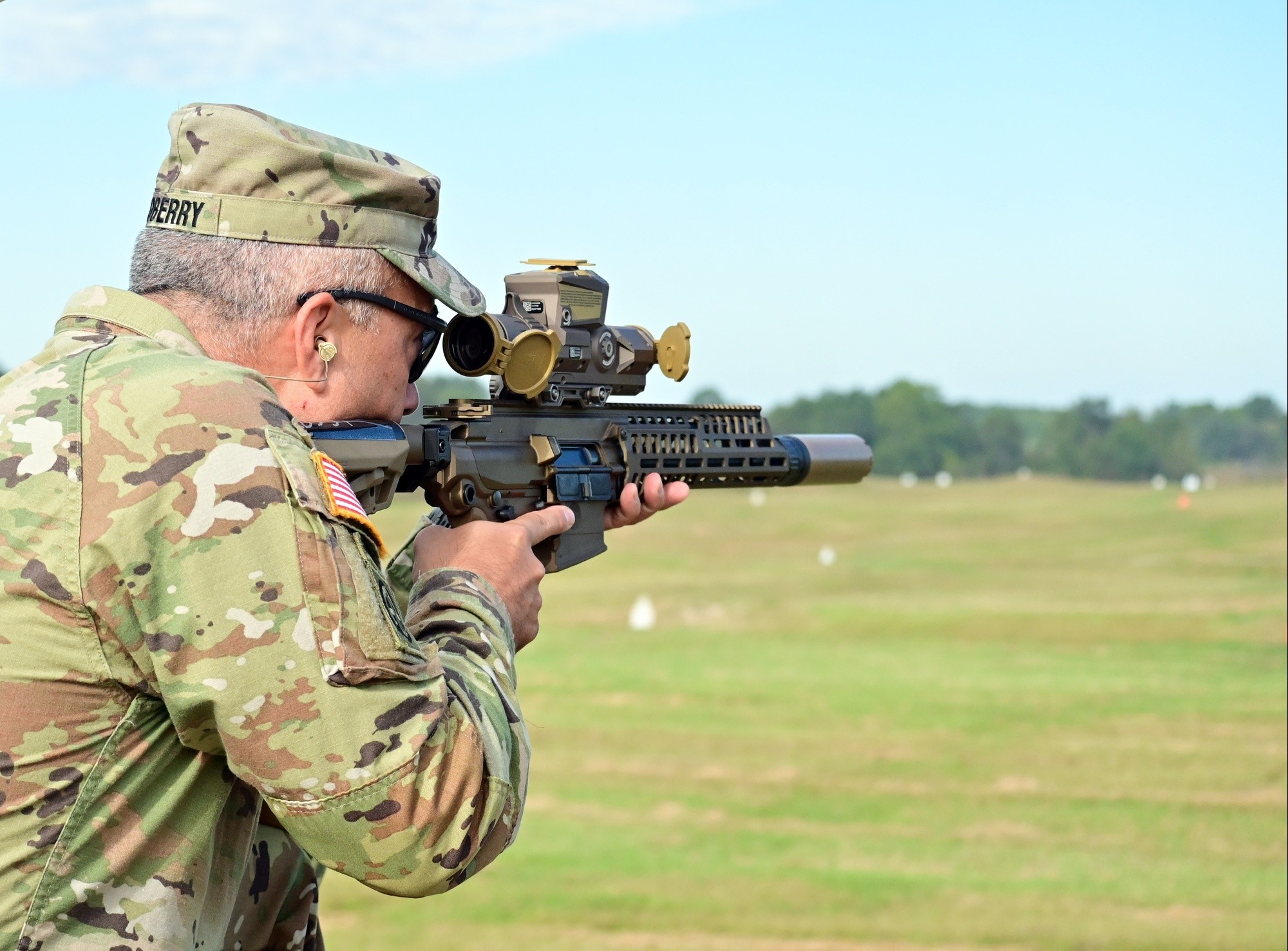In this detailed daytime outdoor image, an older gentleman in full U.S. Army camouflage uniform is the focal point. He stands on the left side of the photograph, aiming a large rifle with a military scope. The uniform, which is a mix of green, brown, dark brown, beige, and tan, features a United States flag patch on his right shoulder, bordered in yellow. He wears sunglasses and a white earpiece, and a military hat with the name "Berry" embroidered in black thread on the back. His gray hair peeks out from under the cap.

The right side of the image shows a green field, peppered with white targets, suggesting a shooting range. Yellow patches of grass hint that it was recently cut. In the distance, rows of trees and possibly a green hill are visible, though blurred. A blue-gray sky stretches across the top of the photograph, completing the serene yet focused atmosphere of the scene.